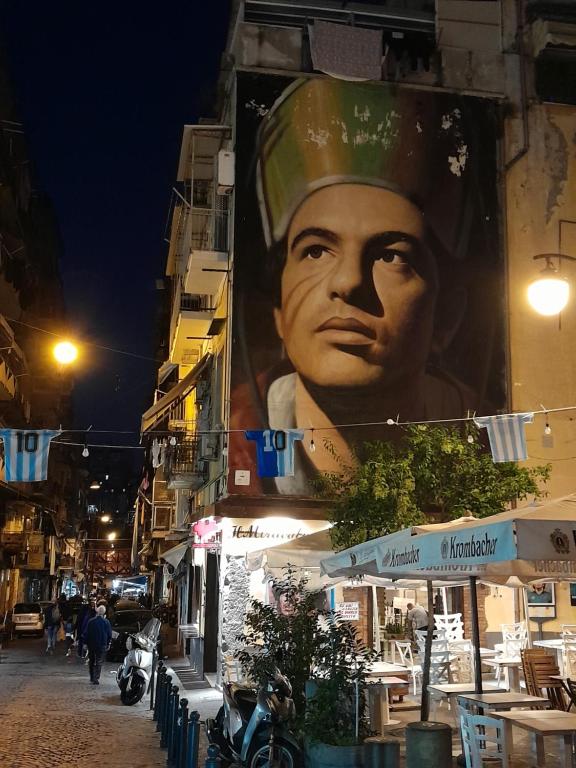This nighttime cityscape photograph showcases a lively yet tranquil urban scene. In the foreground, an outdoor café with white tables and chairs is arranged under tents adorned with advertisements for "Chrome Butcher." Notably, there are no patrons at the café. In front of the café, a motorcycle is propped against a potted plant, adding a touch of casual urban energy. The streetscape includes a few pedestrians strolling down an alleyway that divides the scene, adding a sense of movement and life. On the left side, a second motorcycle and a car are visible, while a strong source of light—likely a streetlight—illuminates this portion of the image, contrasting with the dark blue of the night sky.

Dominating the right side of the photograph, the side wall of a neighboring building features a large, striking poster of a man wearing a greenish-yellow crown and a royal robe, his gaze directed into the distance. This mural adds a regal and somewhat mysterious element to the scene. Above the street, a clothesline stretches across, displaying jerseys emblazoned with the number 10, some in blue and white stripes, others with mixed patterns.

Overall, the image captures a unique blend of urban quietness and hidden vibrancy, from the empty café and parked motorcycles to the distant pedestrians and illuminated artwork.